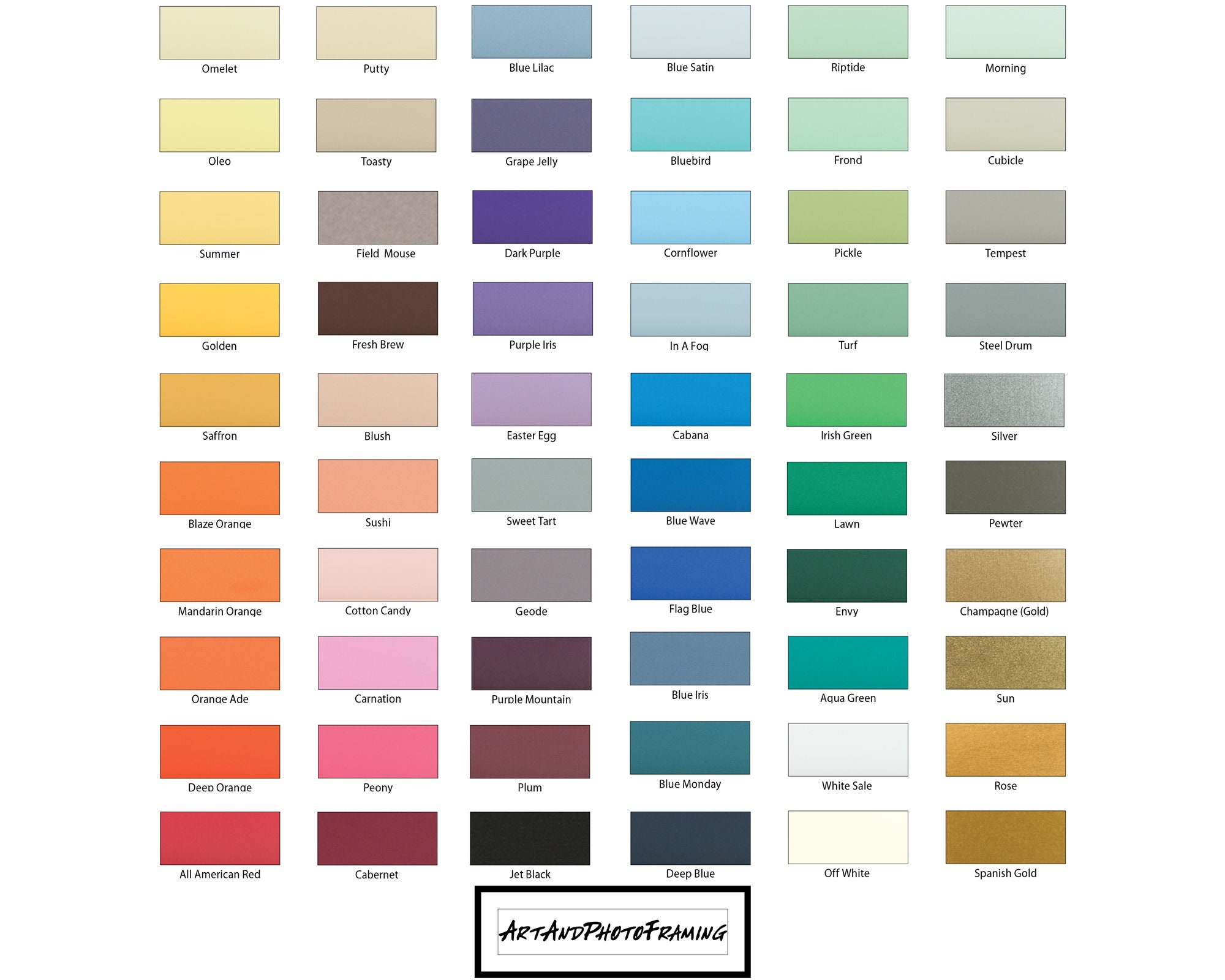The image depicts a detailed color chart against a solid white background, organized into a grid with six horizontally aligned rows and ten vertically aligned columns. Each rectangular swatch is uniquely named and displays a gradient of intensifying tones. The top row transitions from beige through shades of yellow, orange, and red. The second row features a spectrum from beige and gray to pinks and purples. The third row showcases a progression from various blues to deep purples and blacks. The fourth row transitions through a gradient of blues. The fifth row shifts from light to dark greens, ending with whites at the bottom. The final row features a gradient of grays, transitioning into multiple shades of gold. The names of the colors include, but are not limited to, almond omelet, putty, blue lilac, blue satin, riptide, morning, oleo, toasty, grape jelly, bluebird, frond, cubicle, summer, field mouse, dark purple, cornflower, pickle, tempest, golden, fresh brew, purple iris, in a fog, turf, steel drum, saffron, blush, Easter egg, cabana, Irish green, silver, blaze orange, sushi, sweet tart, blue wave, lawn, pewter, mandarin orange, cotton candy, geode, flag blue, envy, champagne gold, orange aid, carnation, purple mountain, blue iris, aqua green, sun, deep orange, peony, plum, blue Monday, white sail, rose, all American red, cabernet, jet black, deep blue, off white, and Spanish gold. At the bottom of the chart, in a black rectangle, is the inscription "Art and Photo Framing."